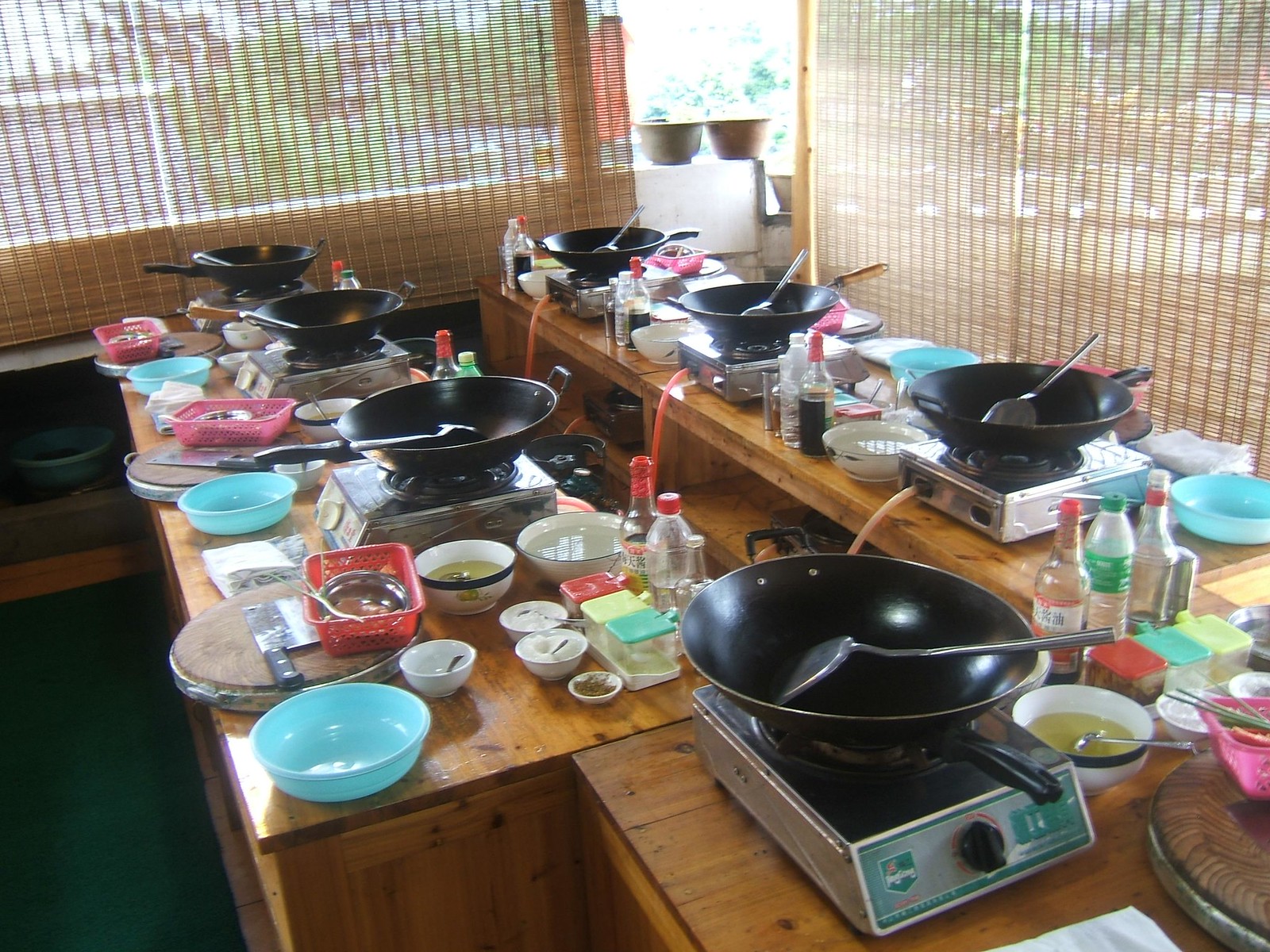The photograph depicts a vibrant and meticulously organized cooking class setup in a room. The main focus is on two long wooden tables and a smaller square table, each equipped with black woks and matching black spatulas placed on electric hot plates. The tables host a variety of items, including assorted colorful bowls—blue, orange, pink, white—filled with an array of cooking ingredients. Visible among these are bottles likely containing oil, soy sauce, rice wine, and various spices. Wooden chopping blocks with knives are also strategically placed at each station.

The countertops, made of a warm brown material, support not only the woks and hot plates but also small bowls and Tupperware-like containers with seasonings. On the background shelves, three hot plates are stacked, each holding additional woks. Surrounding the setup, large windows equipped with rattan-style blinds allow natural light to filter in, with a view extending to a backyard area featuring planters on a ledge. The dark flooring contrasts with the bustling activity of the cooking stations, making the room look ready for a hands-on culinary experience, although no participants are present yet.